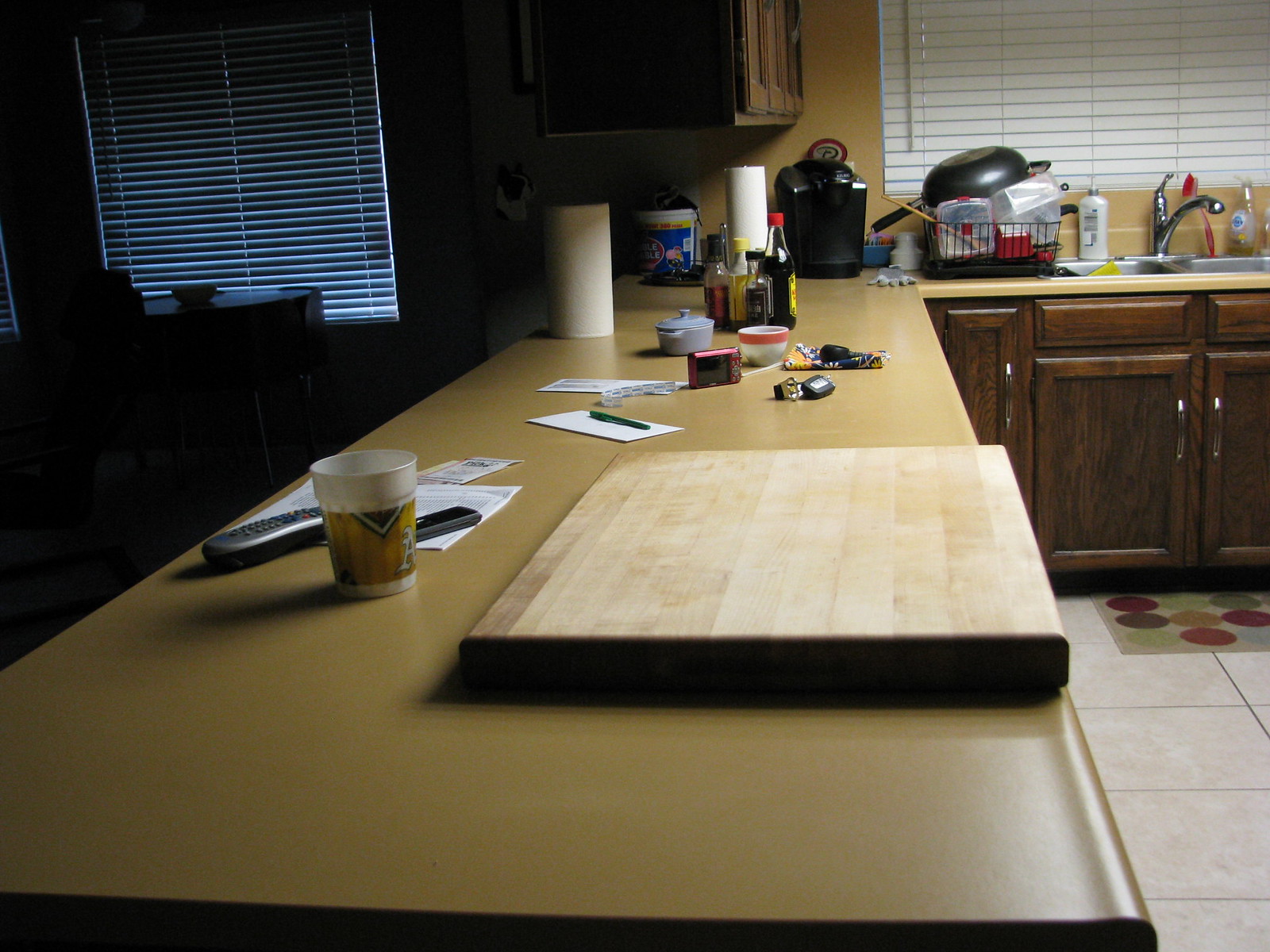In the upper left corner of the image, you can see a series of plastic blinds, predominantly black at the top and lighter in the middle. Adjacent to the blinds is an overhead cabinet. The blinds to the right of the cabinet are fully closed, obstructing the outside light and casting shadows on the left side of the image.

The countertop, primarily brown in color, holds several items. On it lies a brown wooden cutting board and a cup on the left, which features a brown label. A silver controller with buttons rests atop a piece of paper, accompanied by another controller-like device—a thin, black rectangle. Nearby, a white notepad with a pen sits positioned on top. In the background, a red camera is partially visible, revealing its display screen and red metal buttons.

Further right on the countertop, a set of keys lies next to a clock and a coffee cup adorned with a red strand. A stout pot with a lid, a bottle of soy sauce, and a roll of paper towels are also present. A coffee cup can be seen towards the back, near a drying rack that holds various plastic containers and a black pot.

Adjacent to the drying rack is a sink with a silver faucet, which has a white button on the left and a silver button on the right. The under-sink area is flanked by brown wooden cabinets on both sides, each featuring silver handles.

Finally, the floor below showcases a multicolored rug with hues of brown, light green, green, orange, red, and more light green, overlaid on white tile flooring.